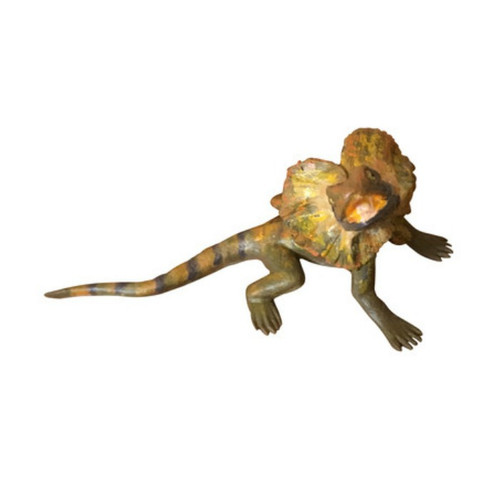This image features a vividly detailed, lifelike toy reptile, resembling a small dragon or dinosaur, displayed against a completely white background. The creature is presented in a dynamic diagonal position, occupying the entire frame with no text or additional elements. Its coloration is a mix of greens, browns, and hints of orange and yellow, predominantly showcasing medium to dark brown shades with distinct dark stripes along the tail. The toy is textured to appear rubbery, adding to its realistic appearance. Positioned with its body towards the three o'clock direction and its head turned towards the viewer, the reptile has its mouth wide open in an aggressive stance, enhanced by two large, intimidating frills reminiscent of a Velociraptor. This central, isolated display suggests a professional photoshoot, likely edited to emphasize the toy, making it a striking and attention-grabbing piece, perfect for a commercial setting like an online toy store.